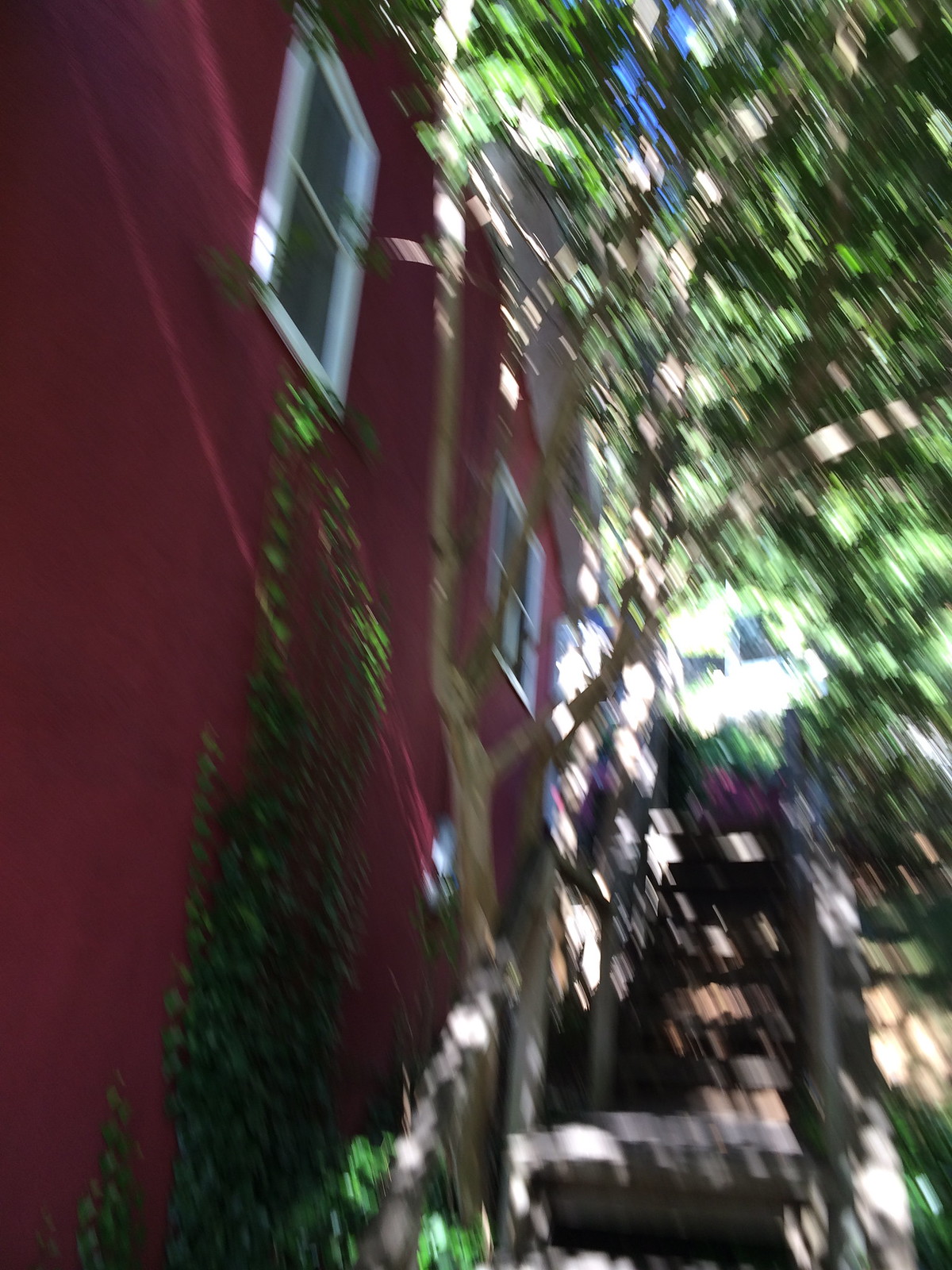This color photograph, though extremely blurry and out of focus, depicts what seems to be a maroon-colored structure on the left side, likely the side of a building. Near the top of the structure, there are a couple of windows with white frames, filled with a featureless gray hue. On the lower right-hand side, there appear to be a few steps, perhaps leading up to a building, characterized by a grayish tone. Furthermore, the upper right-hand corner of the image reveals a significant amount of greenery, suggesting the presence of trees. Additionally, the bright light in this area indicates sunlight filtering through the foliage.